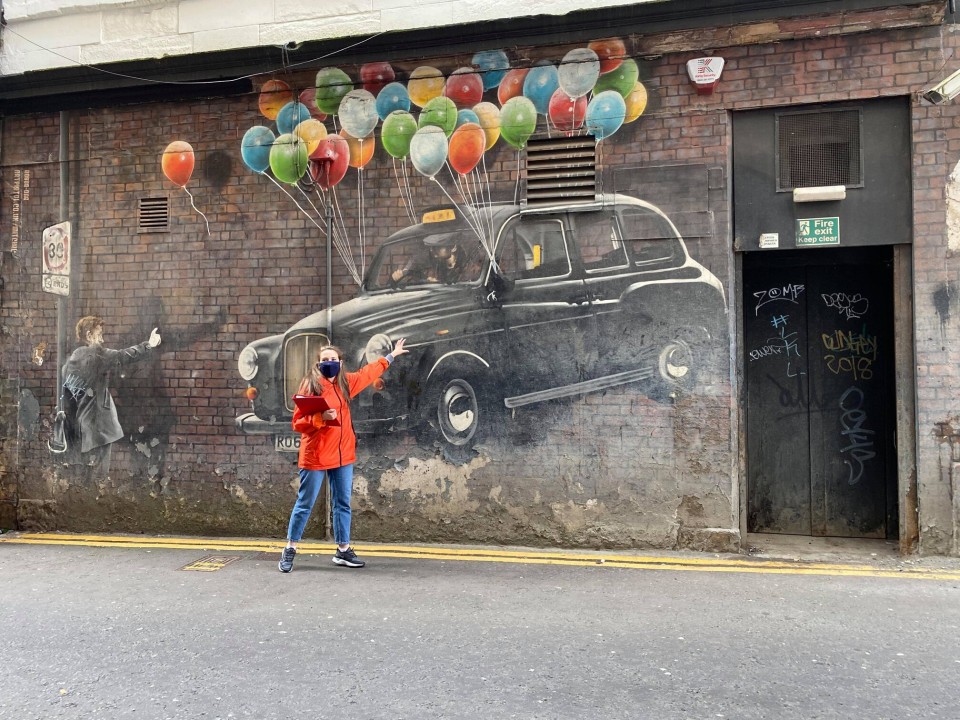This detailed photograph features a vibrant mural painted on a worn brick wall of an old building with graffiti-adorned doors. The mural prominently showcases a vintage taxi cab, reminiscent of the 1940s or 1950s, with a rounded body and gleaming black paint. The car appears to be floating as it is tied to an array of multicolored balloons in primary hues: red, orange, yellow, green, and blue. 

In the mural, a man dressed in a black suit with a shoulder bag is gesturing upwards as if attempting to hail the floating taxi or in awe of the scene. On the left side of the mural, there are street signs and possibly a figure pointing at the car, adding to the narrative element of the artwork.

Standing before the mural is a woman dressed in an orange-red jacket, blue jeans, and black shoes, with a black mask partially covering her face. She is holding a red binder or clipboard and touching the mural with one hand, her pose suggesting an interaction with the art. The street in front of the mural features double yellow lines indicating the center of the road. The setting is urban and dynamic, with the mural adding a lively and imaginative touch to the otherwise aged and graffiti-marked environment.